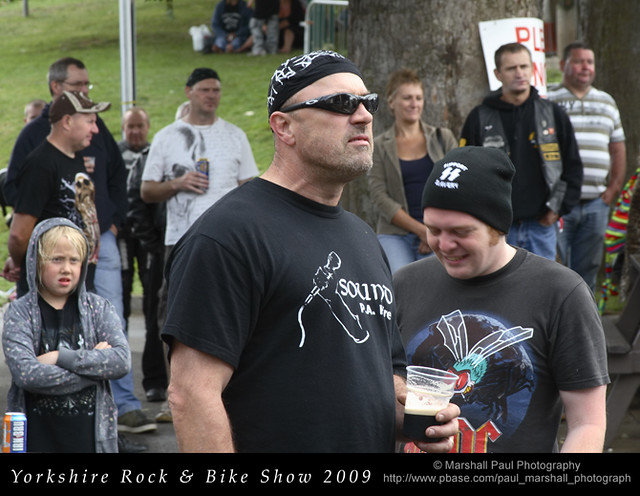In this outdoor image taken at the Yorkshire Rock and Bike Show 2009, the foreground is dominated by an overweight man with an intense expression, wearing a tight black cotton short sleeve shirt, a black cloth beanie resembling a T-shirt texture, and snug sunglasses that are almost goggle-like. His neck vein is prominently visible, emphasizing his anger. He clutches a plastic cup filled with beer, standing out against the blurred crowd around him. There is also a man to his right, who appears to be a boy laughing with his head down, wearing a black woolen cap. Further to the right, behind them, a large tree trunk can be seen with a white sign bearing red lettering, and several people standing next to it. On the left side of the image, a boy with light blonde hair, arms crossed, and wearing a hoodie, appears in the foreground. The scenery extends to a grassy area crowded with people in the background, completing the vibrant, bustling scene.